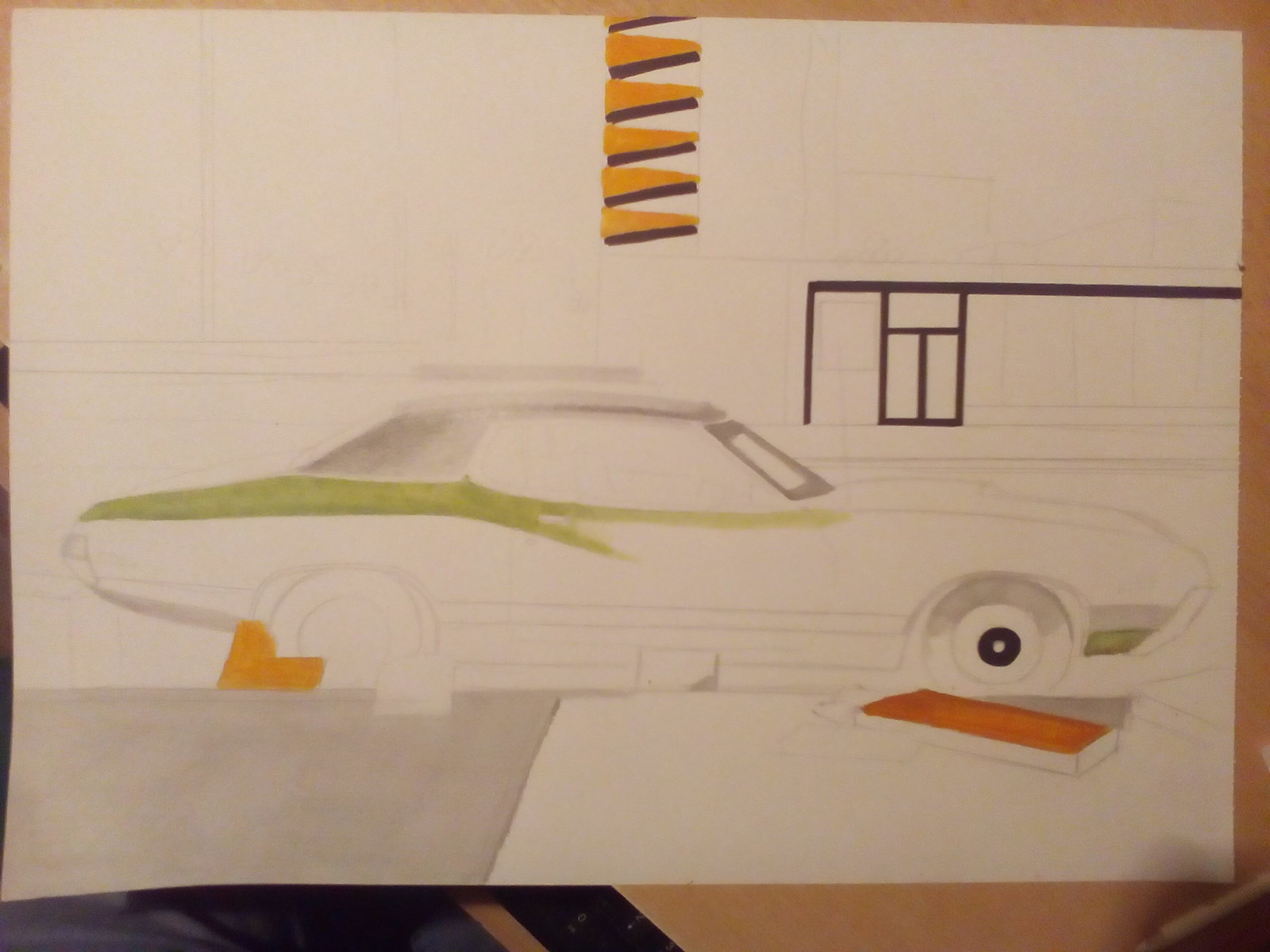An unfinished painting captures the essence of a vintage mid-20th century automobile set against a minimalist, sketched background. The car, meticulously drawn with a striking attention to its sleek, rounded body, remains partially in pencil outline, reflecting the artwork's ongoing progress. Painted sections of the car reveal a primary white hue accented with shades of green and orange, artistically highlighting contours on the hood and intricate elements of the wheel arches. The wheels themselves are partly detailed, showcasing rims and tires in a mix of pencil and paint. The background features simple geometric shapes and lines, hinting at architectural elements like buildings or a garage door, adding context to the elegant vintage vehicle without overpowering the focal subject.